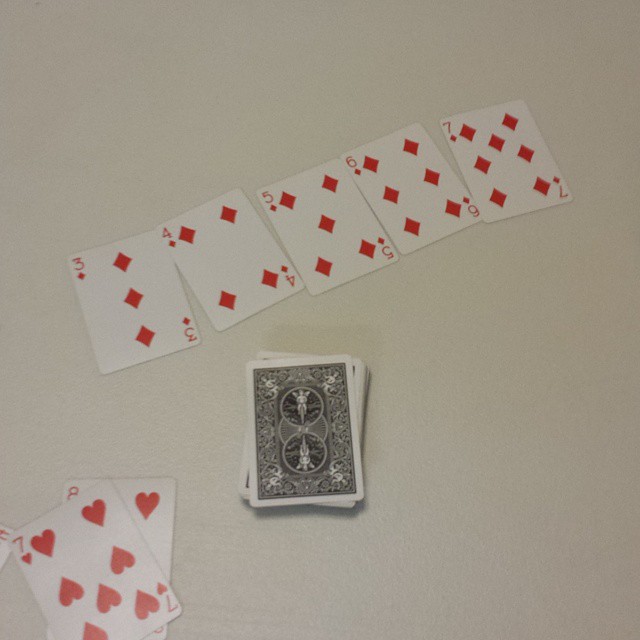The image captures a scene on a white table, prominently featuring a deck of cards placed face down towards the lower part of the frame. Displayed in a linear sequence from left to right are the 3 of diamonds, 4 of diamonds, 5 of diamonds, 6 of diamonds, and 7 of diamonds. Slightly below this linear arrangement, an 8 of hearts is visible, partially overlapped by a 7 of hearts positioned askew, revealing a portion of the underlying card. Additionally, a partial glimpse of another card is visible on the far left edge of the image.

The face-down deck of cards appears substantial and predominantly black with a white trim. The back design showcases a central white angel figure encircled at the top, mirrored symmetrically at the bottom. Additional angels are depicted in each corner, maintaining symmetry whether the card is viewed upright or inverted. The overall composition highlights both the individual details of the cards in play and the ornate design of the deck's backing.